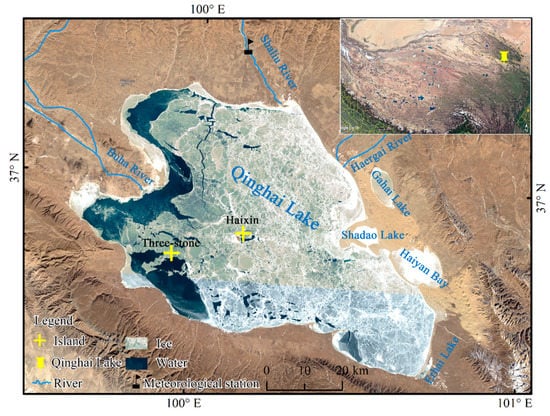This detailed satellite image captures the topography of the area surrounding Qinghai Lake in China, emphasized by its irregular shape and located within a mountainous region. Qinghai Lake is prominently displayed in blue, while adjacent smaller lakes such as Shidao Lake and Gahai Lake, as well as Haiyan Bay, are labeled to the right. The image features a comprehensive legend indicating that islands are marked by yellow crosses or plus signs, rivers are depicted in blue, ice is shown in white, and water is represented by dark blue or black colors. Additionally, the meteorological station is indicated with a black flag. 

A black frame surrounds the entire image, detailing the map's geographical coordinates, with "37 degrees north" marked on both the left and right, and "100 degrees east" and "101 degrees east" labeled at the bottom edges. An inset overview at the top of the image provides a broader perspective of the region. 

This vibrant map utilizes a palette of blues, silvers, tans, and a bit of green, with text labels primarily in blue and the legend in black font. There is also an overlay likely added for enhanced detail, including labels for landmarks like the Hergai River and various roads.